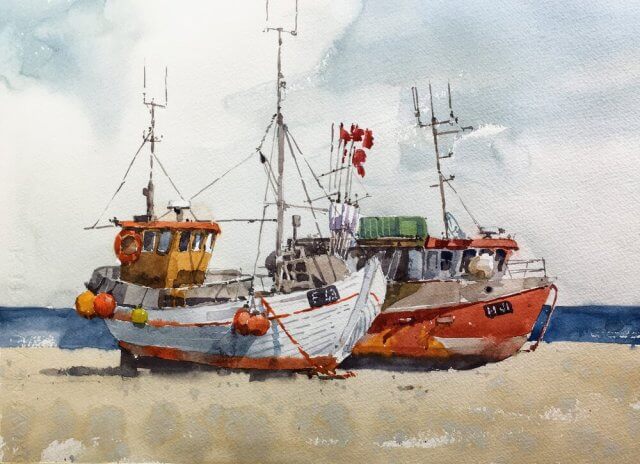This watercolor painting vividly depicts two distinct fishing boats docked on a brown sandy beach, set against a backdrop of a bright blue ocean and a light blue-gray sky. The boat on the left is predominantly white and smaller in size, featuring a yellow captain's section and orange and yellow buoys hanging off its sides. The boat on the right is a copper-red color with a larger crew area, where a few more people could presumably stand or sit. It also has a green object atop the cabin and, like its counterpart, sports a tall, though currently unattached, sail. Both boats are equipped with antennas on their cabins and appear to have signs on them, adding to the detailed charm of this coastal scene.